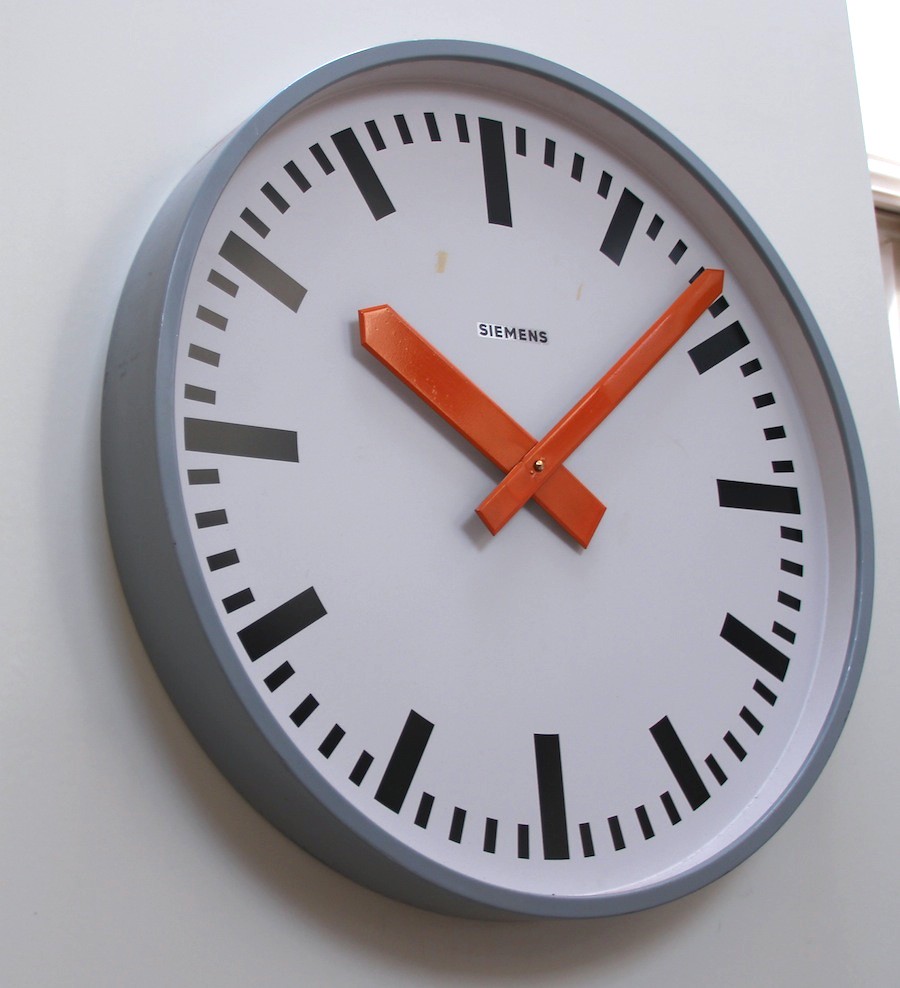The image features a sleek, modern wall clock prominently displayed on a stark white wall. The clock, which appears to be constructed from metal, is encircled by a gray border that provides a crisp contrast against its white face. The clock's hands, vibrant in red, stand out distinctly and indicate the time as 11:09. The brand name "Siemens" is clearly visible on the clock's face, adding a touch of sophistication. Uniquely, the clock features thick black vertical lines marking the hours, with shorter black lines denoting the minutes, instead of traditional numerals. The clock is positioned near the edge of the wall, revealing a glimpse of the adjoining room to the right side of the image, enhancing the scene's depth and context.